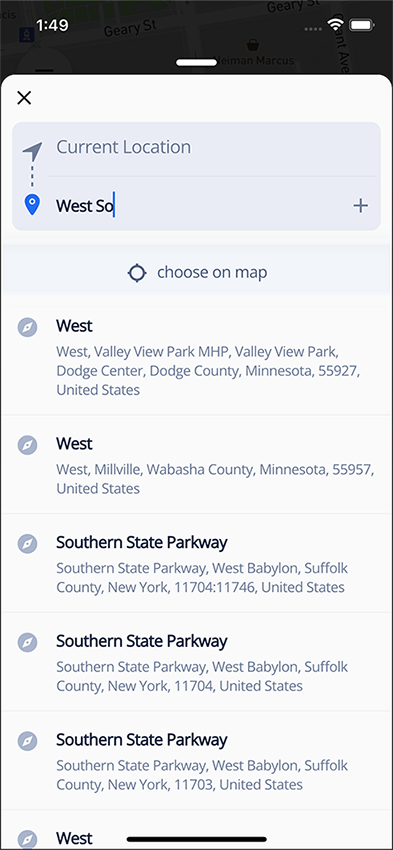This image is a screenshot featuring a predominantly gray background. The display shows a digital time of 1:49. At the upper left corner, it lists "X current location" and "West SO." In the center, a blue cursor indicates that the user is actively typing. There is also a plus sign next to an option labeled "Choose on map."

The mid-section of the screenshot contains location information in a well-organized format. It lists 'West Valley View Park, MHP' in all capital letters, followed by:

- Valley View Park, Dodge Center, Dodge County, Minnesota, 55927, United States
- West Millville, Wabasha County, Minnesota, 55957, United States
- Southern State Parkway, West Babylon, Suffolk County, New York, 11704, 11746, United States
- Southern State Parkway, West Babylon, Suffolk County, New York, 11703, 11704, United States (Repeated entries for locations on Southern State Parkway)

At the bottom middle of the screen, there is a prominent black bar stretching across.